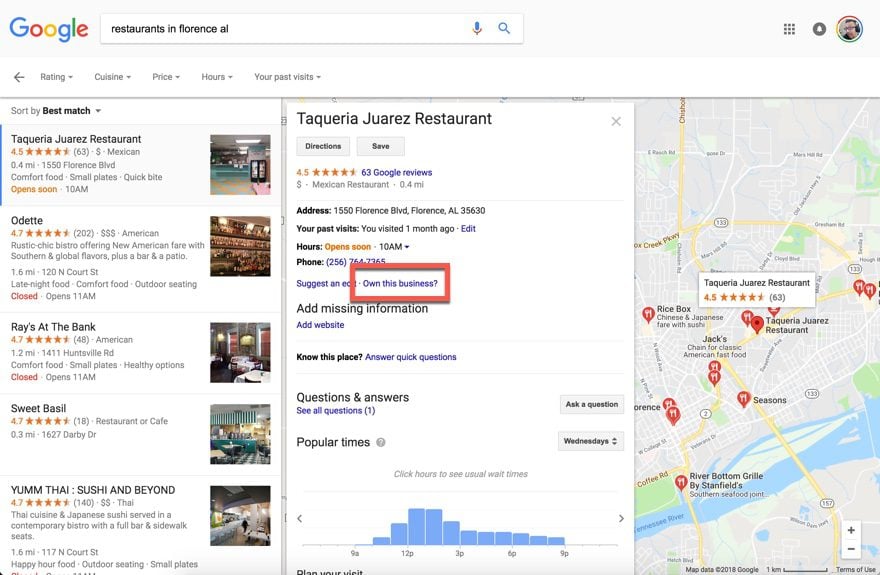Screenshot of a Google search for "restaurants in Florence, AL." At the top, the Google logo in its signature colors (blue, red, yellow, green) is displayed next to a search bar containing the query. Icons for a microphone and magnifying glass are adjacent to the search bar. The top-right corner features a grid of nine circles and a user avatar within a multi-colored border.

Below, navigation arrows and drop-down menus labeled "Rating," "Cuisine," "Price," "Hours," and "Your past visits" are visible. The left section lists several restaurants: "Taqueria Juarez Restaurant," "Odette," "Ray's at the Bank," "Sweet Basil," and "Yum Thai Sushi & Beyond." Each entry includes the restaurant's distance, star rating, and a thumbnail image of its interior.

The main focus is on "Taqueria Juarez Restaurant," showing detailed information: 4 out of 5 stars from 63 Google reviews, address (1550 Florence Boulevard, Florence, AL 35630), business hours (opening at 10 a.m.), a partially obscured contact number, and a "Suggest an edit" link. A red banner labeled "Own this business" is present, along with options to add missing information, website, and answer quick questions.

Further down, a "Questions and Answers" section includes a button to ask a question, and a "Popular Times" graph indicates peak hours from 12 p.m. to 3 p.m. The map on the right displays a grayscale layout with red pinpoints marking locations, highlighting Taqueria Juarez Restaurant with a 4.5-star rating.